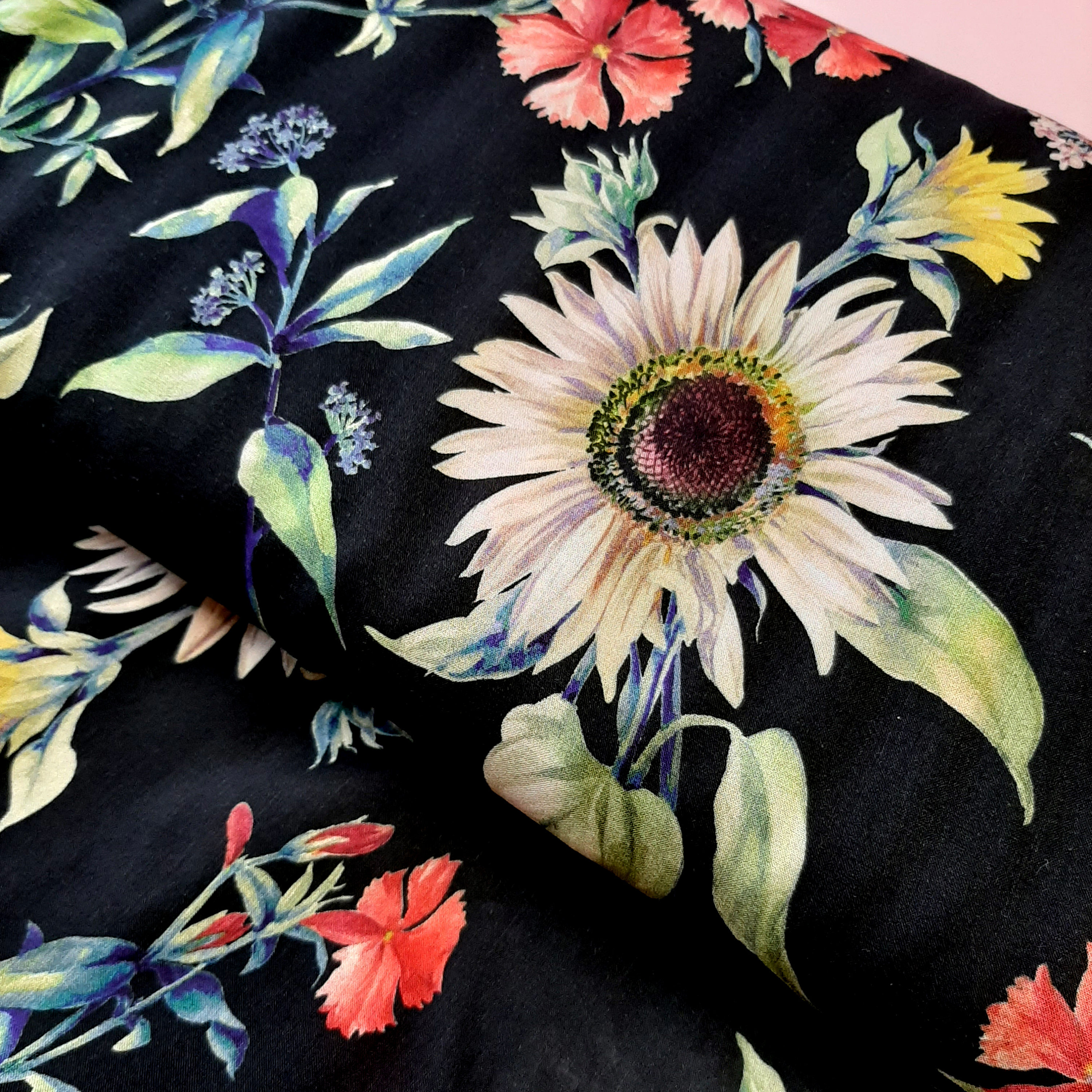This image features a detailed photo of a black fabric, likely resembling a blanket or another type of textile material with a soft, velvety texture. The fabric is adorned with an array of vivid, colorful floral patterns. Central to the design is a large white flower, akin to a sunflower, with a pinkish, almost rainbow-like glimmering center encircled by green leaves. Surrounding this prominent bloom, various other flowers are artistically arranged, including vibrant pink, red, blue, and yellow blossoms. 

In particular, small coral flowers can be seen scattered towards the corners and the center of the pattern. The upper left corner is graced with delicate baby's breath-like flowers alongside additional greenery, adding to the intricate botanical motif. The textured black background amplifies the vibrancy of the flowers, making them stand out. The overall appearance suggests it could be a roll of fabric, a pillowcase, or a blanket, presenting a visually rich and tactilely inviting piece of fabric art.